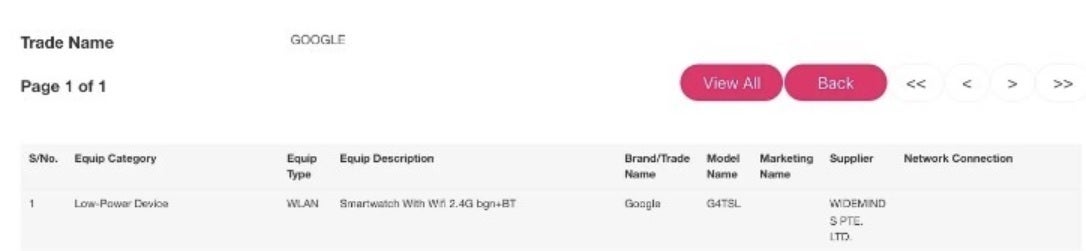This image is a web screenshot detailing the specifications of a piece of equipment. The top left corner features the text "Trade Name" in bold, and directly beneath it, the label "Page 1 of 1." To the right of "Trade Name," the word "GOOGLE" appears in all caps and black font. 

The next section, titled "Equipment Category," lists the category as "Low Power Device," and the "Equipment Type" is identified as "WLAN." Following this, there is an "Equipment Description" that specifies the item as a "Smartwatch with 2.4G."

Further details include:
- Brand: Google
- Model: G4TSL
- Supplier: Widowed SPT ELTD

These details are displayed within a light gray rectangle, using black font. The text on the top row of this rectangle is bolded, while the bottom-row text is not.

At the top of the interface, there are three buttons positioned in a horizontal line. The leftmost button is a long oval with flat top and bottom edges, rounded sides, and a pink background. It has white text that reads "View All." 

Adjacent to this is an identical button that says "Back" in white text. To the right of these buttons are navigation arrows: a set of two arrows pointing left, a single arrow pointing left, a single arrow pointing right, and a set of two arrows pointing right.

The website's background is white, and all the text throughout is in black. The "Trade Name" text is in bold, as is the top row of text on the light gray rectangle, while the remaining text is not bolded.